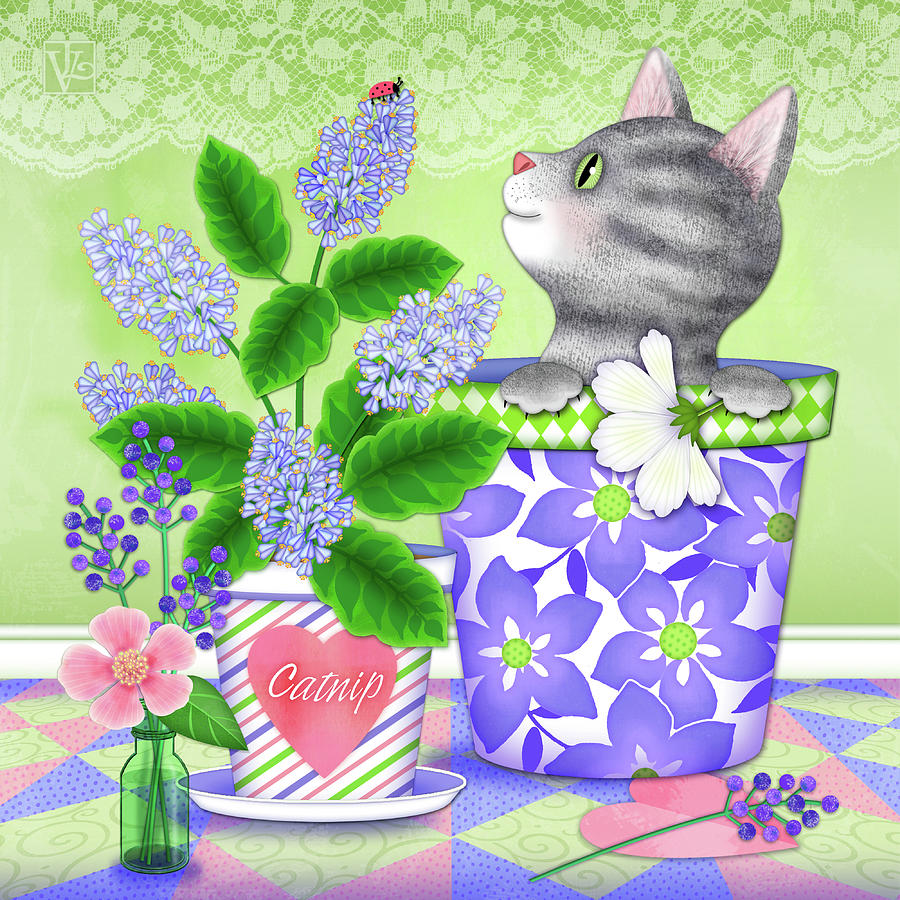In this vibrant and playful illustration, a gray cat with mesmerizing green eyes is depicted peeking out of a uniquely decorated flower pot, which is adorned with violet floral designs. The cat, appearing curious and serene, holds a delicate white flower in its paws and gazes upwards, seemingly engaged in a whimsical interaction with a ladybug hovering above. The background is a striking lime green, embellished with an intricate floral lace pattern at the top and a stylized logo featuring an upside-down 'A' and an 'L'. The floor beneath the pot is equally colorful, featuring alternating hues of green, pink, and purple with polka dots, diamonds, swirls, and heart motifs. To the left of the cat, there is another flower pot bearing an image of a heart printed alongside the word "catnip," filled with a lush plant. A small, charming vase containing additional flowers and a tiny plant also sits nearby, adding to the enchanting garden-like setting.